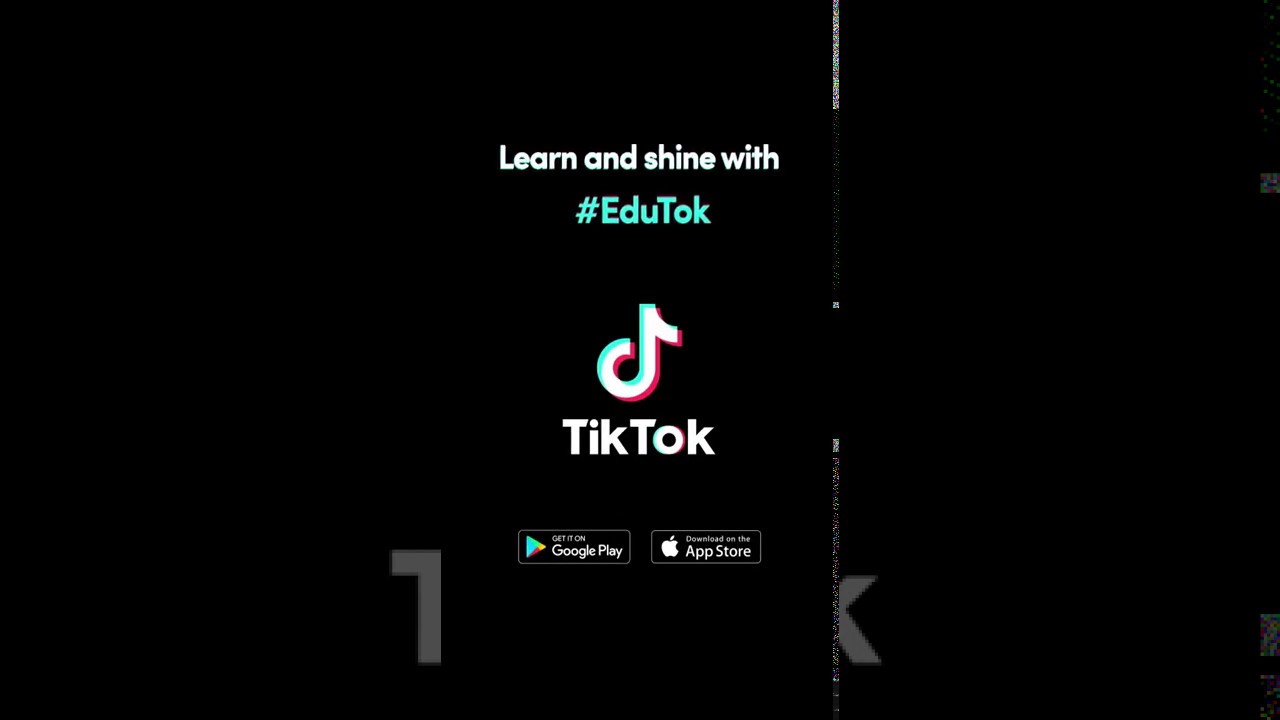The image features a predominantly solid black background, with a notable area of intricate detail in the bottom right-hand corner. Upon close inspection, this corner reveals an array of colors, including green, yellow, and red, forming a rectangle. These colors continue upward, culminating in speckles at the top right-hand corner.

Centrally positioned on the image is the text "LEARN AND SHINE WITH" in bold white, uppercase letters. Beneath this, a row of text in a light teal color reads "#EDUTOK" next to the distinctive TikTok logo, which blends teal, white, and a pinkish-red.

Directly beneath this row, the word "TikTok" appears in white, aligned below the logo. Adjacent to this, on the left and right sides, are two black rectangles with white borders. The rectangle on the left displays the Apple logo accompanied by the phrase "Download on the App Store." The rectangle on the right features the Google Play logo, a triangle composed of green, blue, yellow, and red colors, alongside the text "Get it on Google Play."